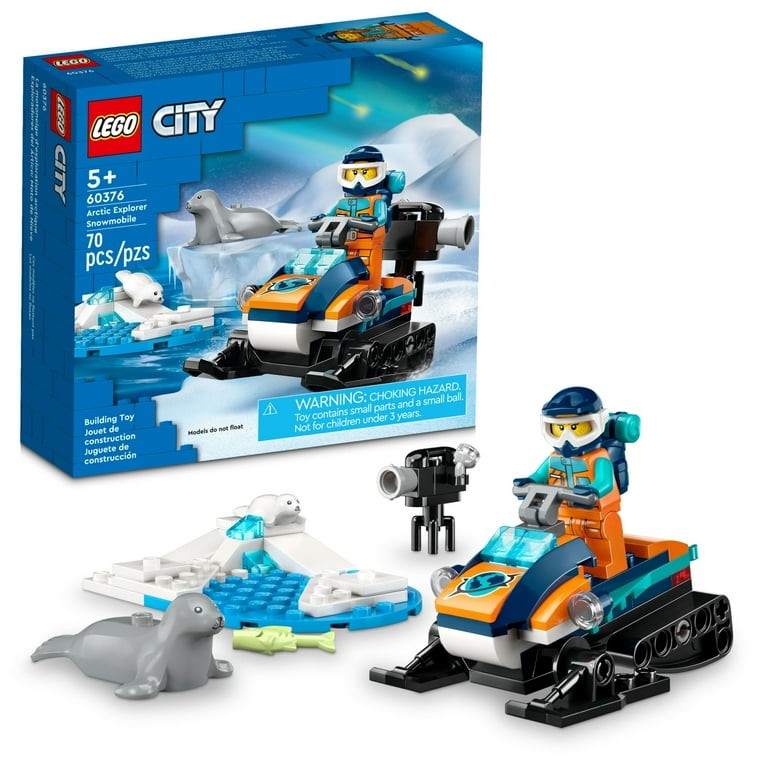The image showcases a detailed Lego City Arctic Explorer Snowmobile set, designed for children aged 5 and up. The blue packaging prominently displays the Lego City logo and a vivid scene of a Lego character riding an orange and blue snowmobile over a snowy landscape, complete with shooting stars in the sky. The set includes an array of accessories and characters, such as a polar bear, two seals with flippers spread out, and a camera. The bottom of the box features a clear illustration of all included pieces, which total 70 items, alongside a warning for small parts. Bright turquoise blue accents highlight important information, including the age recommendation and potential choking hazards.